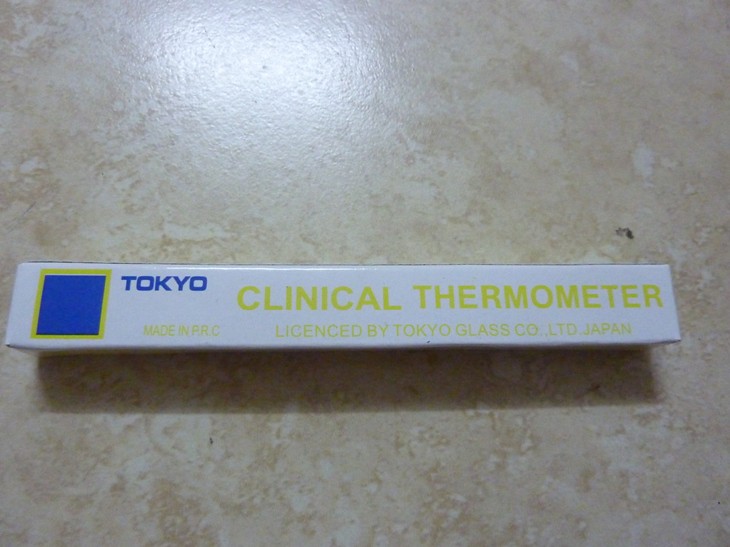This vertical color photograph captures a pristine cardboard box neatly placed on a table. The box, which is white, prominently displays a logo with the word "Tokyo" in blue. Surrounding this blue box is a lime green outline, while the rest of the text on the box is also in lime green. The product inside is identified as a "Clinical Thermometer." The box states that this thermometer is made in PRC (People's Republic of China) and is licensed by Tokyo Glass Company, LTD, Japan. The table on which the box rests appears to be a laminate surface, featuring a blend of beige tones intermixed with light beige and white swirls. A light source illuminates the table, casting a gentle shine across the surface. The box remains unopened and retains its fresh, untouched appearance.